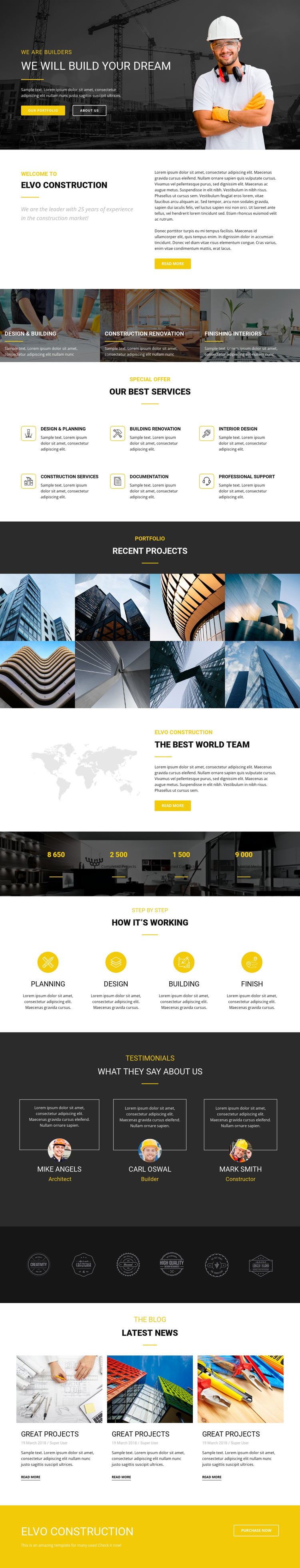The image is a detailed screenshot from the homepage of the Elvo Construction website. At the top, there is a black banner displaying various construction tools alongside a construction worker outfitted with full safety gear—helmet, goggles, noise-canceling headphones, and gloves. The banner features the text "We are builders. We will build your dream" in bold, with a bright yellow banner reading "Our Portfolio" underneath it in white print.

Below the banner, there is a white-outlined square labeled "About Us" which introduces Elvo Construction, spelled as E-L-V-O. The section provides a background and details about the company's history and services.

As you scroll down, a graphic illustrates a range of their expertise with categories like "Design and Building," "Construction," "Renovation," "Finishing and Interiors." Accompanying this, a highlighted area presents a "Special Offer: Best Services," listing out offerings such as "Design and Planning," "Construction Services," "Building Renovation," "Documentation," "Interior Design," and "Professional Support."

Further down, the "Portfolio" section showcases recent projects with various designs and constructions. There's also a map with a tagline stating "Elvo Construction: The Best World Team."

Towards the bottom, a step-by-step guide is provided detailing their process: Planning, Design, Building, Finish, and Test. The testimonials section highlights "What They Say About Us" with various customer reviews. Finally, the blog section titled "Latest News" features repeated mention of "Great Projects."

Overall, the website conveys a comprehensive look at Elvo Construction's services, showcasing their portfolio, client testimonials, and detailed information about their process and expertise.